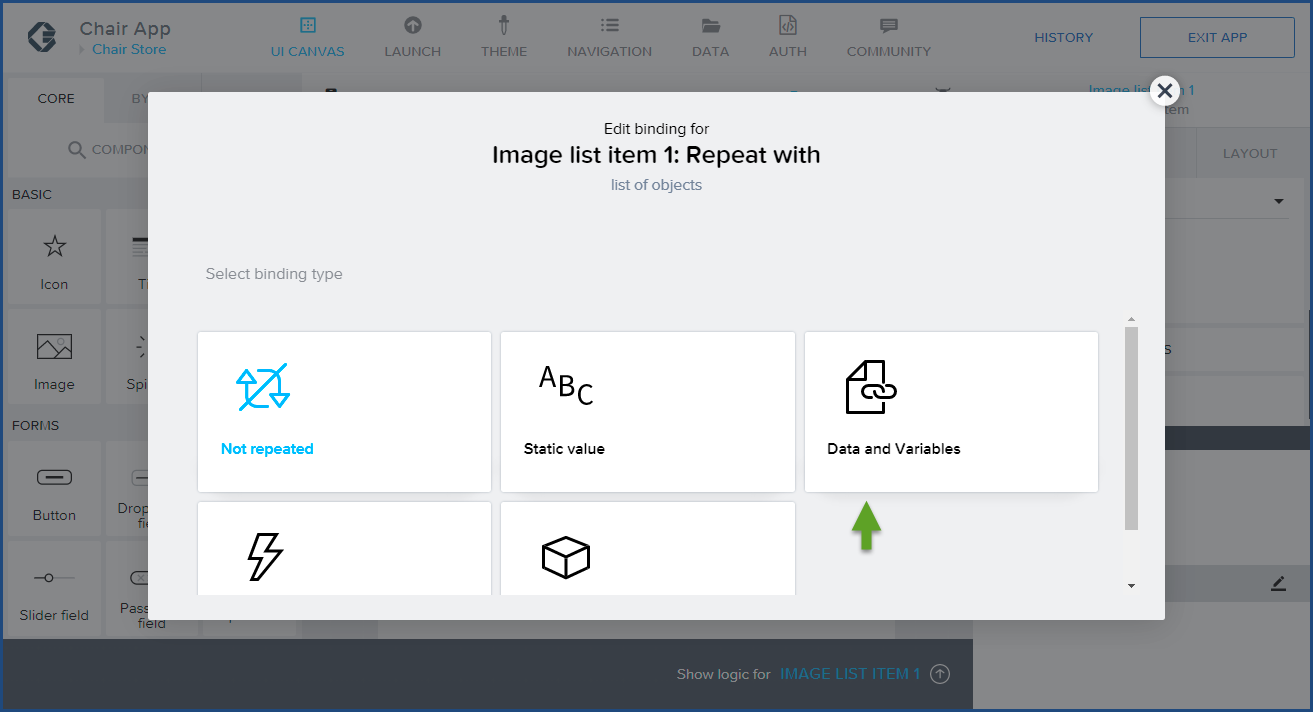The image depicts a webpage with an active pop-up window, which appears to be a configuration or editing interface for an application. The pop-up window is titled "Edit Binding," and lists a series of editable parameters. At the top of the window, text reads "Image List Item 1." Below, a dropdown menu displays an option labeled "Repeat with," followed by another dropdown reading "List of Objects." Further down, the section "Binding Type" is accompanied by several selectable options: a square icon with two arrows crossing through, labeled "Not Repeated," an "ABC" icon for "Static Value," and another option marked "Data and Variables."

Behind the pop-up, the background webpage showcases the user interface of an application described as "Chair App" and "Chair Store," with these titles located at the top-left corner. Adjacent to these titles, several interface buttons are visible: "UI Canvas," "Launch Theme," "Navigation," "Data," and "Authorized Community." To the right of these are buttons labeled "History" and "Exit App." 

Below the main navigation bar, partially obscured by the pop-up, are additional categories titled "Basic" and "Forms," under which appear to be more selectable options or clickable boxes, suggesting further configuration or form fields related to the app's functionality.